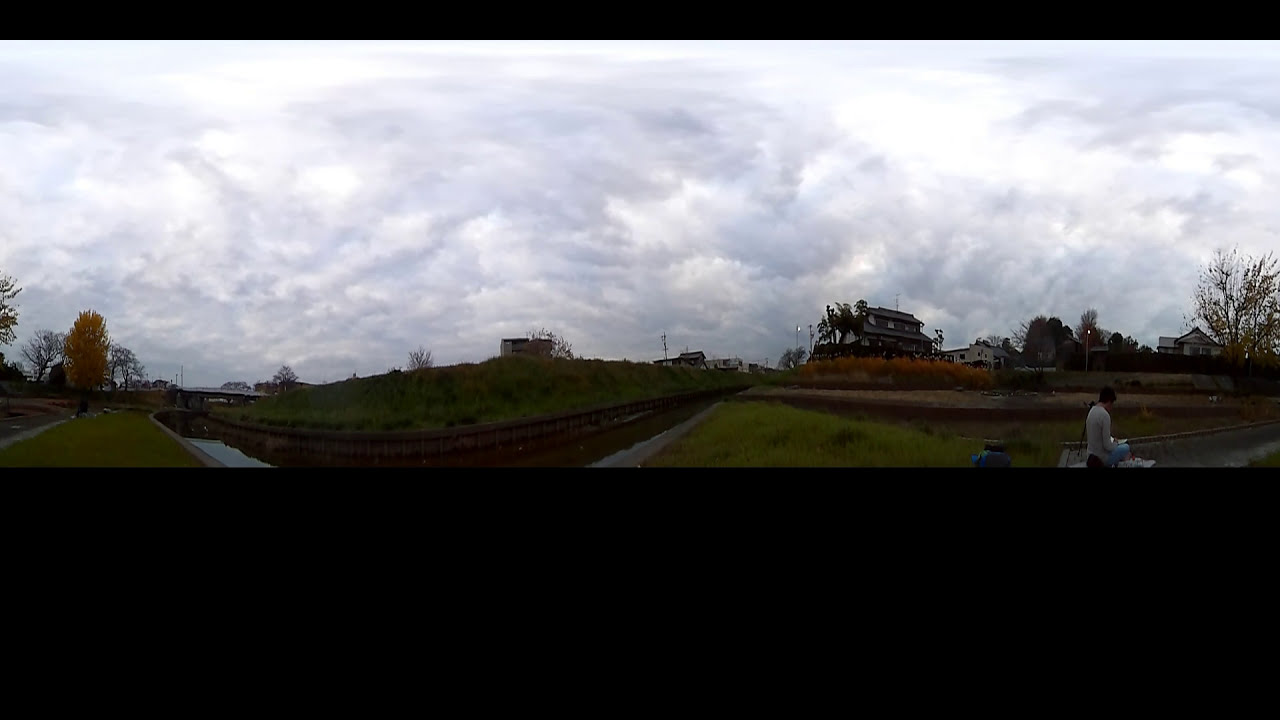The image depicts a serene countryside scene dominated by a heavily clouded sky. Thick, light to dark gray, puffy clouds roll and curve into each other, creating an impressive and beautiful backdrop with no blue sky visible. The photograph spans a wide horizontal frame with thin black lines bordering the top and the bottom, partially obscuring the lower portion of the image. 

In the foreground on the right side, there is a person wearing blue trousers, a gray sweater, and a mauve backpack. The person is standing, possibly on a bench or stool, and appears to be gazing thoughtfully at the cloudy sky. The landscape features lush green grass and numerous trees scattered throughout. A water canal weaves through the middle distance, curving gracefully and disappearing towards the left. In the far background, one can make out a few distant buildings and houses, adding a quiet, homely feel to the scene. There might be a river or lake surrounded by greenery, further enhancing the tranquility of the countryside setting.